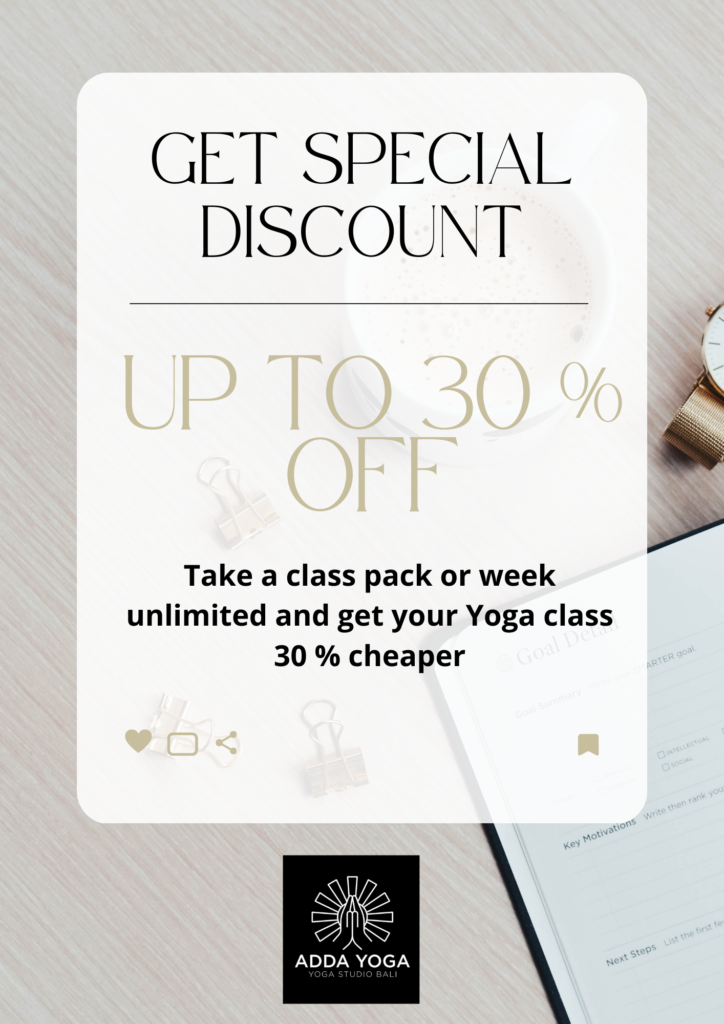This vertical image, likely intended as an advertisement for discounts, features a visually appealing layout against a wooden desk or table background. The light brown and white grains and lines of the wood are clearly visible, adding a natural and warm aesthetic. On the right-hand side of the image, a gold and white clock is partially visible, along with an open booklet titled "Key Motivations, Next Steps, Goals," designed for jotting down personal notes or objectives.

Centrally placed is a long rectangular box with rounded edges, colored in black. The text inside the box is prominently displayed in uppercase letters that read "GET SPECIAL DISCOUNT." Below this bold invitation, a thin black line divides the text from further details written in a tan color, also in uppercase, stating "UP TO 30% OFF." Additional bold black text elaborates on the offer: "Take a class pack or week unlimited and get your yoga class 30% cheaper."

At the bottom of the image, a row of icons resembling heart favorites, sharing, and bookmark tabs can be seen, suggesting options for user interaction. Just beneath these icons, a small black square contains a white icon, and accompanying text that reads "ADDA Yoga."

Overall, the image effectively combines informative text with appealing design elements to advertise a compelling yoga class discount.